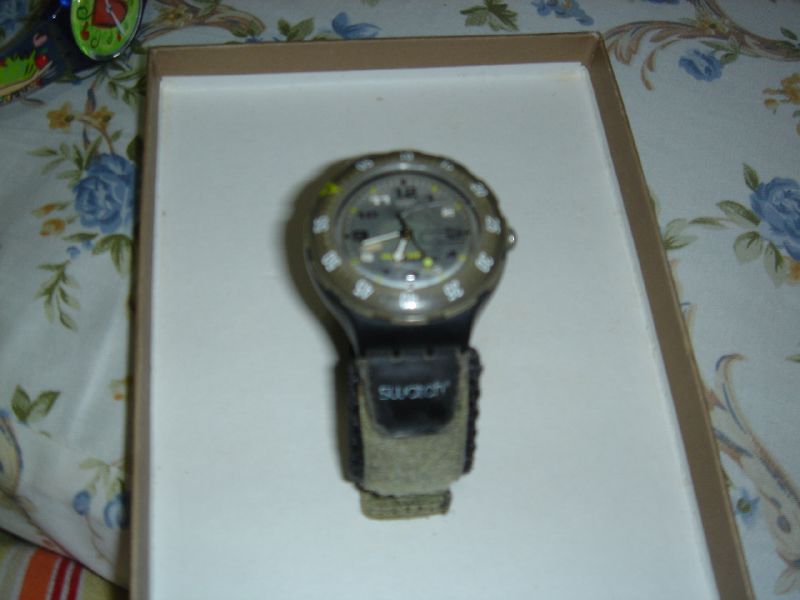This photograph captures a detailed and somewhat cluttered scene featuring a bulky, rugged gold Swatch sports watch prominently placed in the center. The watch, which has an outer metal bezel with minute markers ranging from 25 to 60, is positioned on the inside of an upturned box lid, which appears to be from a pair of trainers due to its white interior and gold exterior. The inner watch face is grey, displaying traditional numbers from 1 to 12, with white hour and minute hands and a black second hand showing a time of approximately 6:42. The watch has a Velcro strap, which is gray with black accents and partially folded beneath it, revealing the Swatch branding.

The box lid occupies most of the image but is cut off at the bottom edge, and it rests on a bedspread adorned with blue and green flowers. Additionally, a small part of another watch with a luminous green face, red center, and black strap is visible in the top right corner, though it is partially out of frame. The overall scene also includes elements of a children’s toy in the bottom left, contributing to the image's eclectic arrangement.